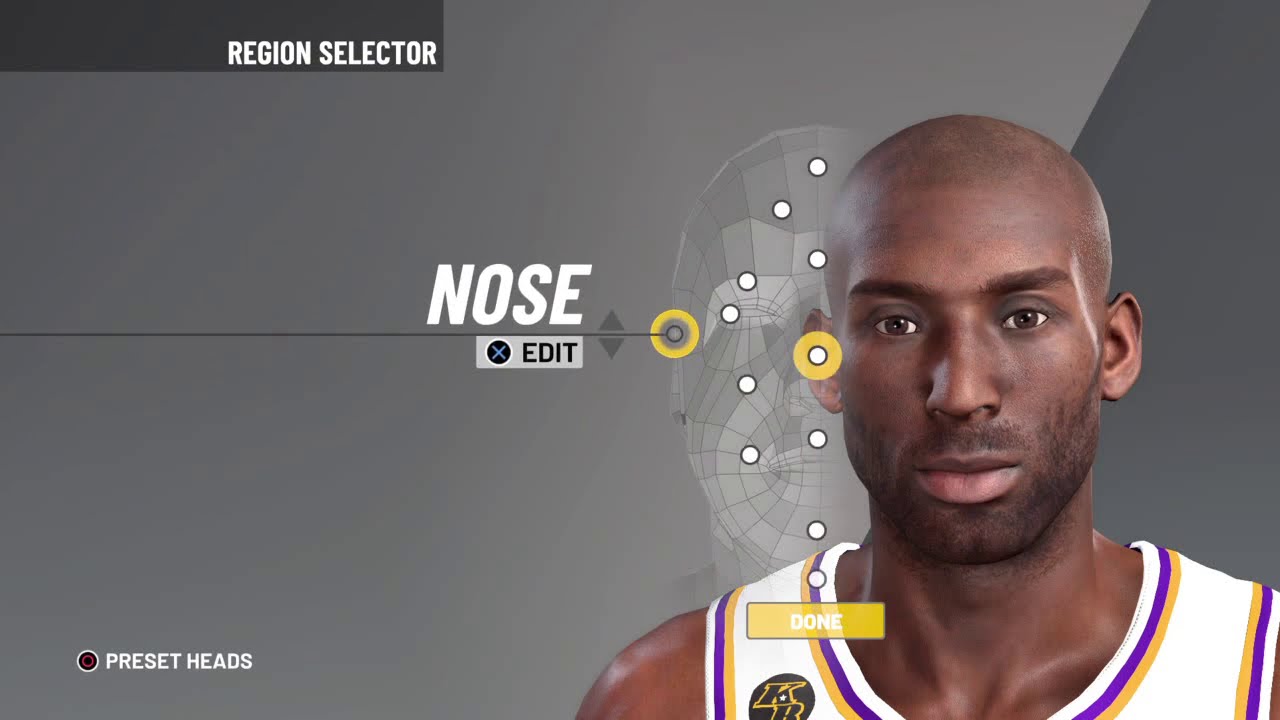In this image, we see a gray-themed room consistent with a game character creation screen. The upper left corner features a darker gray banner labeled "Region Selector", with options for "Nose" and "Edit" visibly highlighted. The focus is on a virtual avatar, which is modeled after the late NBA star Kobe Bryant. This avatar is donning a white LA Lakers uniform, trimmed with purple and gold accents. The screen currently allows players to modify the nose of the character, showcasing the advanced customization options available. This detailed and interactive interface reflects the remarkable technological advancements in gaming, allowing users to create highly personalized avatars, albeit raising questions about the allocation of such technology.